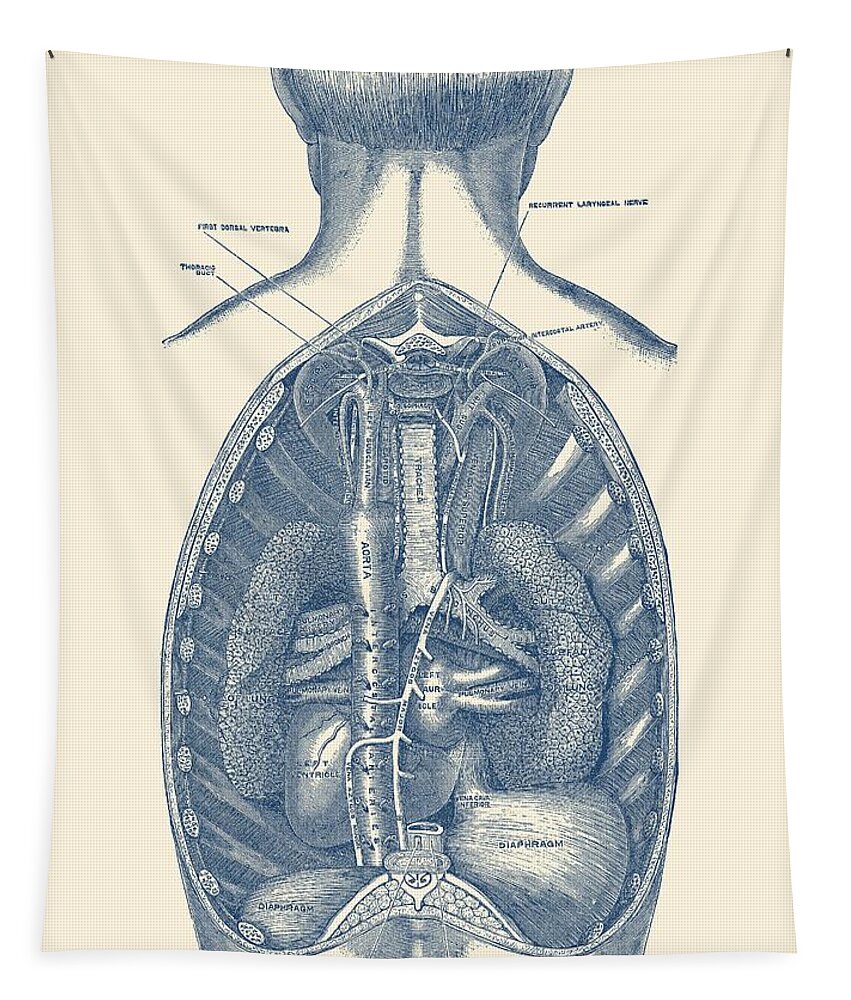The image depicts a detailed, black and white artistic representation of the back of a human anatomy, printed on a cloth-like fabric with a slight pinkish hue. The fabric is vertically rectangular and is attached to a wall using two stick pins at the upper corners. In the illustration, the back of a man's head is visible, showing his hair, parts of his ears, neck, and upper shoulders. Below this, the skin is split open to reveal the internal organs, focusing on the thoracic and upper abdominal regions. This comprehensive anatomical study includes visible ribs, lungs, heart, liver, kidneys, and other major organs. Lines extend from various points to tiny text labels that identify these organs; however, the writing is very small and difficult to read. Some labels mention "diaphragm" and "recruitment latitudinal nerve." The overall impression is that of an educational diagram designed to provide a thorough view of the male internal anatomy from a dorsal perspective.